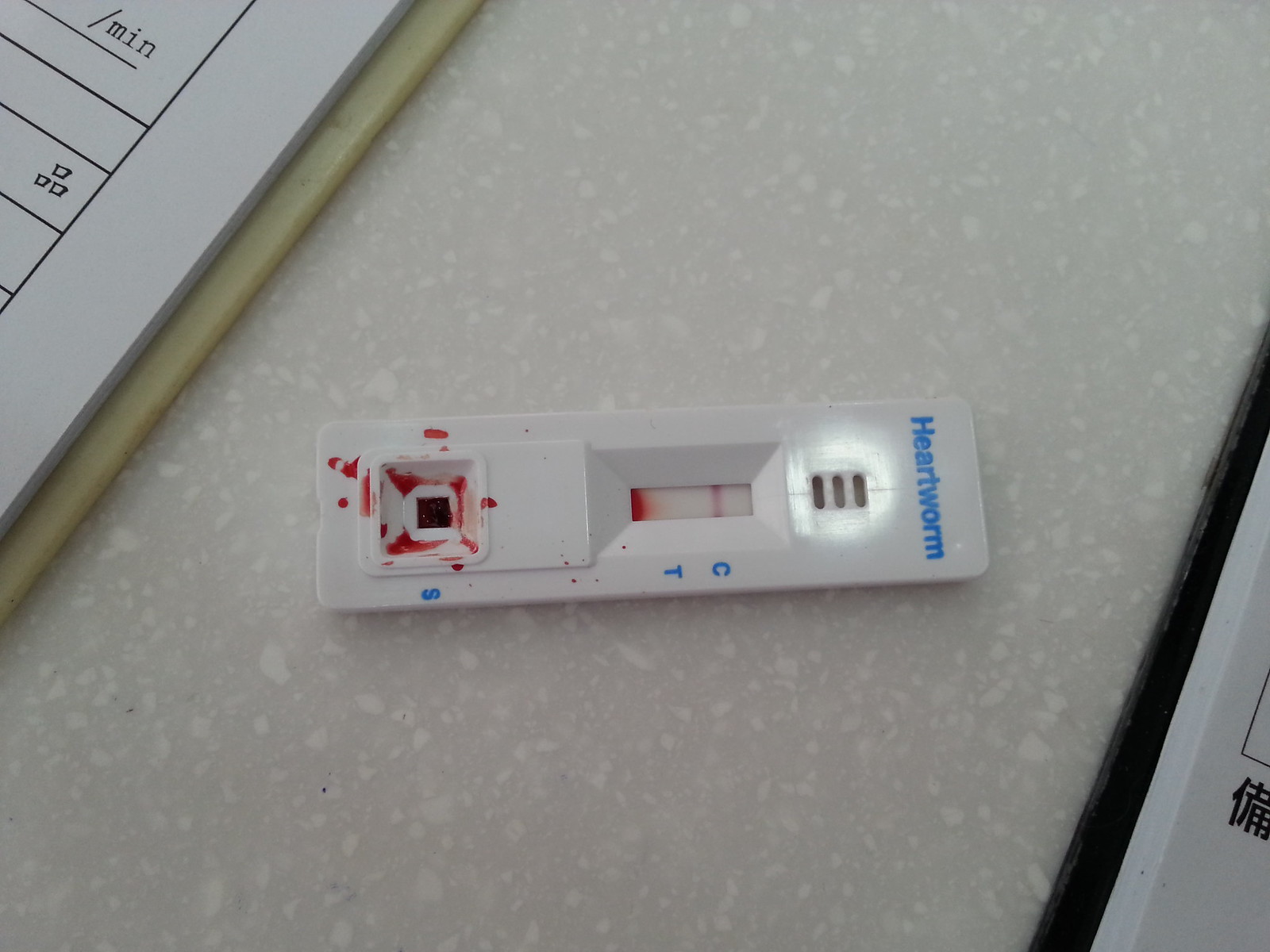A close-up image of a heartworm test kit is depicted. The test kit, resembling a COVID-19 test, is primarily white and rectangular with the label "Heartworm" printed in blue. It features an area marked "CNT," likely indicating control and test sections. The sample area, denoted by a blue "S," is visibly contaminated with blood. The blood is present not only within the sample square but also along the edges and speckling the surrounding area. The test kit rests on a white, speckled surface. Additionally, a notepad with a partially visible clipboard and the text "/MIN" in black can be seen in the corner of the photo.